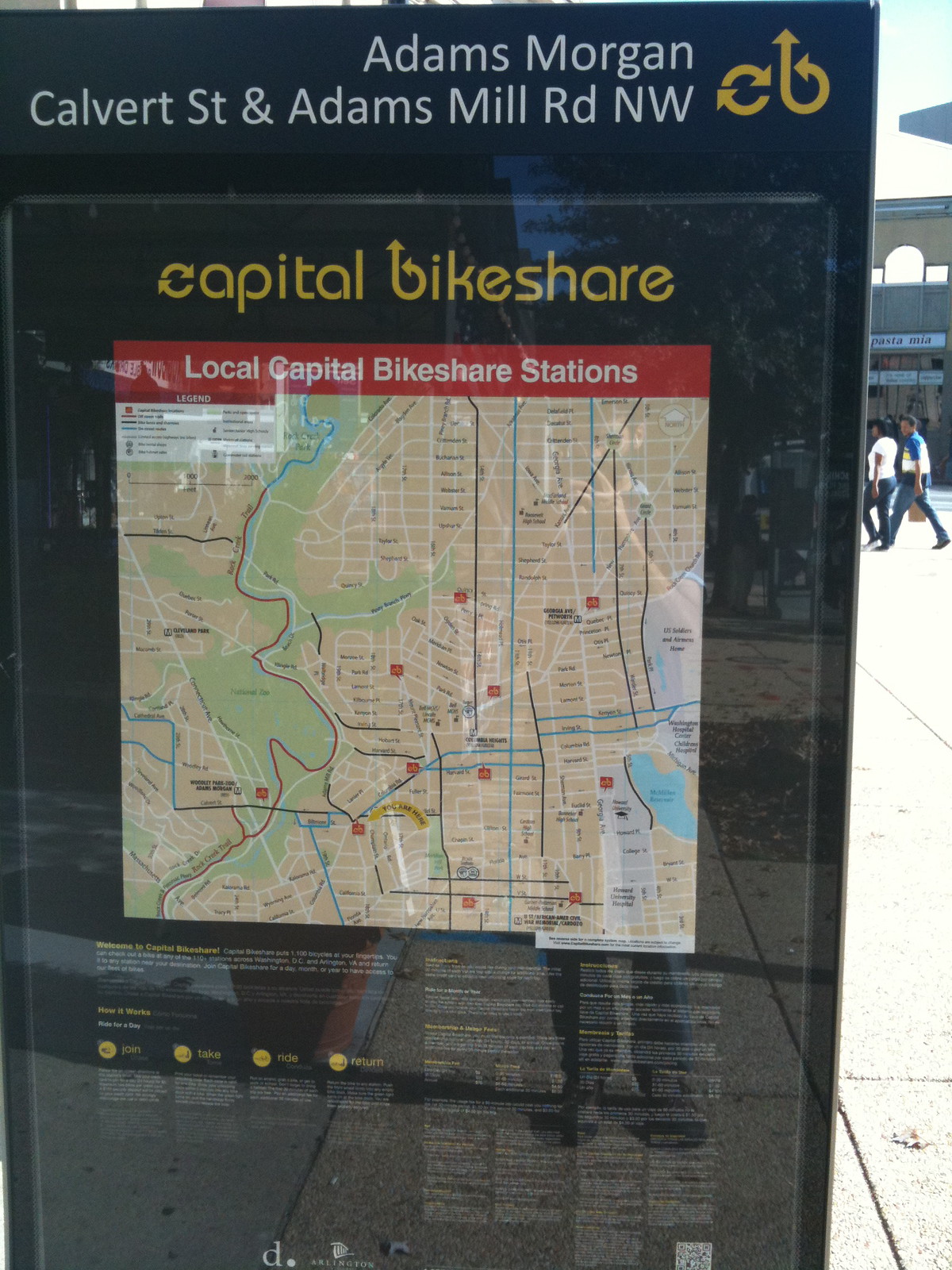The image depicts a highly reflective, glass-encased, black sign positioned on a sidewalk or street, as indicated by the surrounding gray stone pavement. The sign is set against a backdrop of a brightly lit, daytime urban environment, with people walking and buildings visible. At the top of the sign, in bold white letters, it reads: "Adams Morgan, Calvert Street, and Adams Mill Road, NW." Below this header are three golden arrows pointing in different directions: up, right, and left.

Prominently featured in the center of the sign is the Capital Bikeshare logo followed by the text "Local Capital Bikeshare Stations" highlighted in red. Beneath this title, a map predominantly colored in beige and light green displays various black, blue, and white lines, along with several icons indicating the locations of Capital Bikeshare stations. The map includes a QR code in the bottom right corner and is surrounded by numerous icons and text.

The lower section of the sign contains detailed instructions and information, including phrases like "Welcome to Capital Bikeshare, Join, Take, Ride, Return." Additionally, the reflection on the sign reveals the legs of the person taking the photo, adding to the reflective quality of the glass. Overall, the sign provides comprehensive guidance for users of the bikeshare program and integrates seamlessly into its urban surroundings.